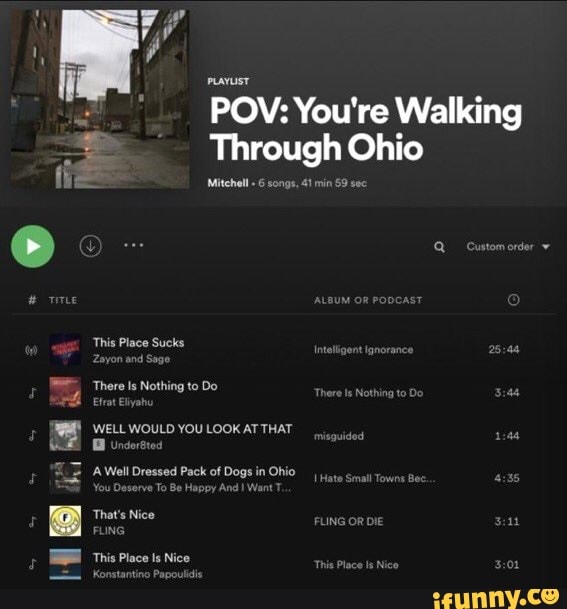Title: "Mitchell's Ohio Walk-Through Playlist"

Caption: 
Immerse yourself in a unique auditory experience with Mitchell's curated playlist titled "This Place Sucks, There is Nothing to Do." This captivating 6-song compilation, lasting 41 minutes and 59 seconds, offers a point-of-view walk through the nuanced landscapes of Ohio, presented via a visually engaging video on iFunny.co. The somber backdrop features a charcoal black theme, setting a moody ambiance perfect for the reflective journey.

The playlist thumbnails depict various scenes and thematic titles, including "Well, Would You Look at That" and "A Well-Dressed Pack of Dogs in Ohio," juxtaposing elements of the mundane with the unexpectedly delightful. The overall visual design exudes an urban vibe, with a gray sky evocative of an overcast dawn or dusk, post-rain stillness more commonly found in an industrial area.

Highlights of the imagery include occasional street lamps casting their light on puddles reflecting the muted sky, intertwined with high-rise buildings and utility poles adorned with wires, epitomizing the quintessential urban street scene. The play button, distinguished by its green color, is strategically positioned towards the upper left, inviting viewers to embark on this auditory exploration of Ohio's urban charm and understated allure.